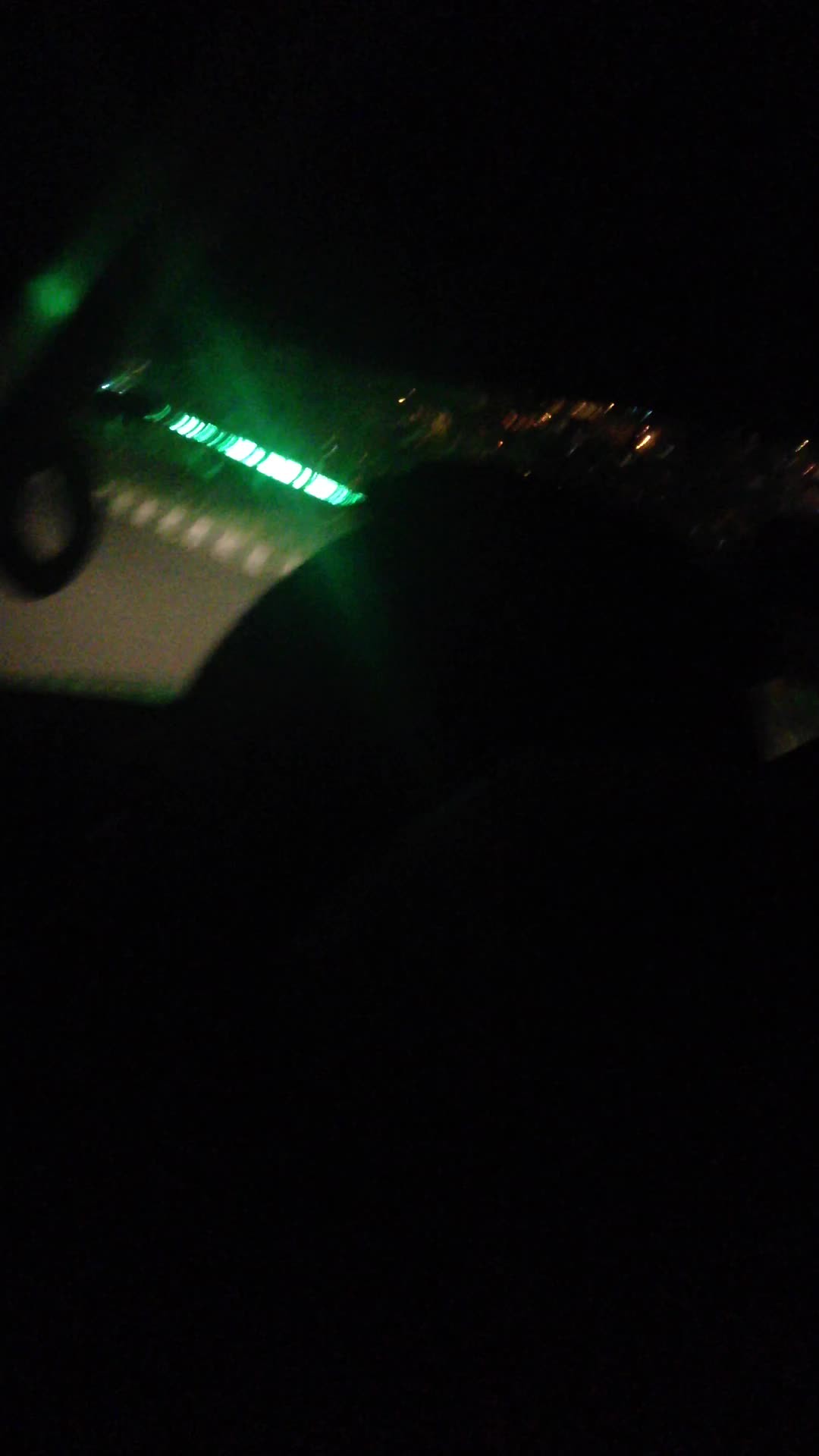This photograph, taken in portrait mode, captures a very dark and dimly lit scene, likely from inside a car, possibly from the back seat. Dominating the bottom right to the middle of the image is a nearly black silhouette, possibly of a seat back, with a slight curved shadow along its surface. In the center left, there's a black circular object, possibly a steering wheel, enhancing the impression that the photo was taken from a vehicle's interior. Through what seems to be a windshield, a street is visible, indicated by faint white lines suggesting a crosswalk. One of the most prominent features is a series of neon green lights glowing on the side of the road, possibly displaying words, though they are unreadable. Above these green lights are some yellow lights, which might be from houses on a hill. Additionally, there appears to be some reflections, possibly water droplets, on the windshield, catching light and adding to the scene's ambiance. Despite the overall darkness of the image, these illuminated details stand out, giving the photograph a mysterious nocturnal quality.